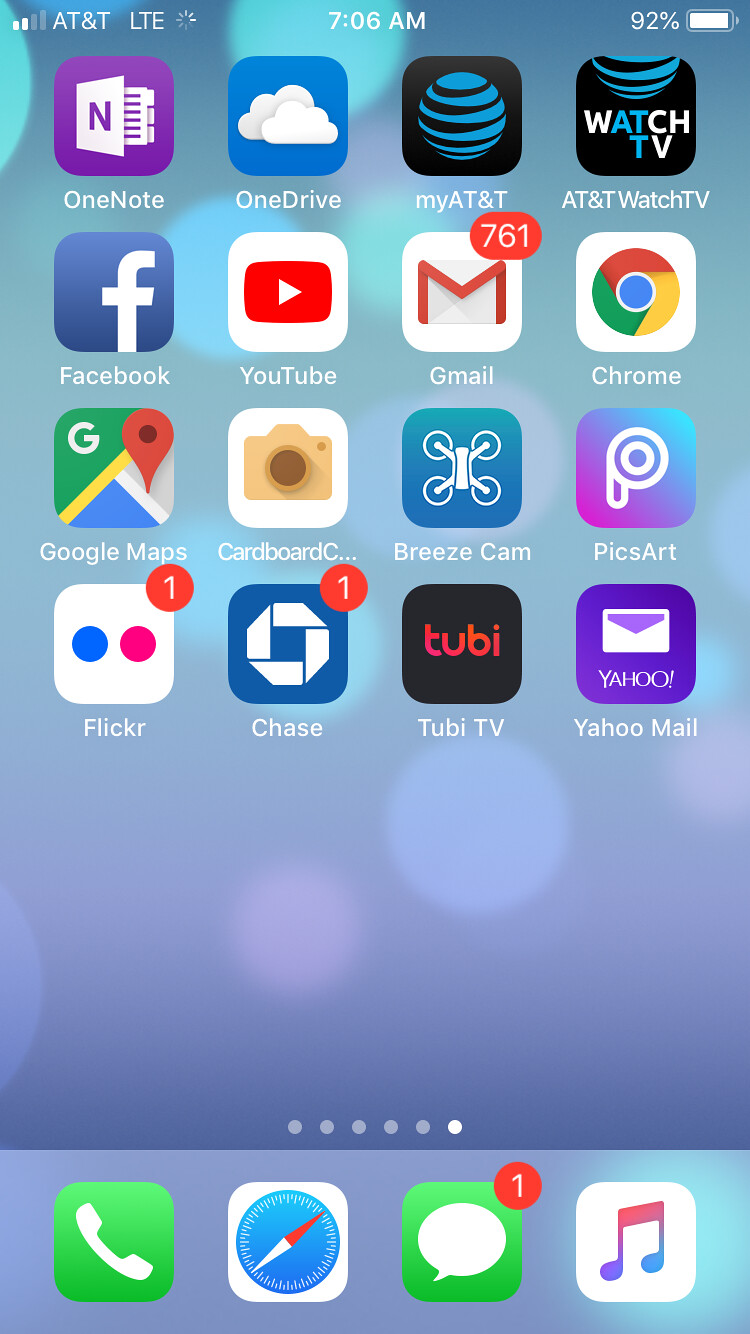This image showcases an Apple iPhone screen featuring a well-organized grid of app icons against a soothing, gradient background. The background transitions from lighter to darker shades of blue, embellished with subtle, out-of-focus circular bubbles giving it a serene, dreamy appearance.

The app icons are arranged in a neat 4x4 grid:
- **Top Row (left to right):** OneNote, OneDrive, MyAT&T, AT&T WatchTV
- **Second Row:** Facebook, YouTube, Gmail, Chrome
- **Third Row:** Google Maps, Cardboard, C, BreezeCam, Pixar
- **Fourth Row:** Flickr, Chase, TubiTV, Yahoo Mail

Additionally, there's a persistent row of heavily used app icons at the bottom:
- **Phone App:** Green phone icon.
- **Safari:** Compass icon.
- **Messages:** Speech bubble icon with a small red notification badge displaying the number one.
- **Apple Music/iTunes:** Musical note icon.

At the top of the screen, you can see the essential status icons:
- **Service Bars:** Only two bars filled, indicating a modest signal strength.
- **Carrier & Network:** AT&T LTE, accompanied by a small loading symbol.
- **Time:** Displayed centrally at 7:06 AM.
- **Battery Status:** Showing 92% with the battery icon nearly full.

This detailed layout provides a clear and comprehensive view of the user’s device screen, highlighting both the functional and aesthetic elements.